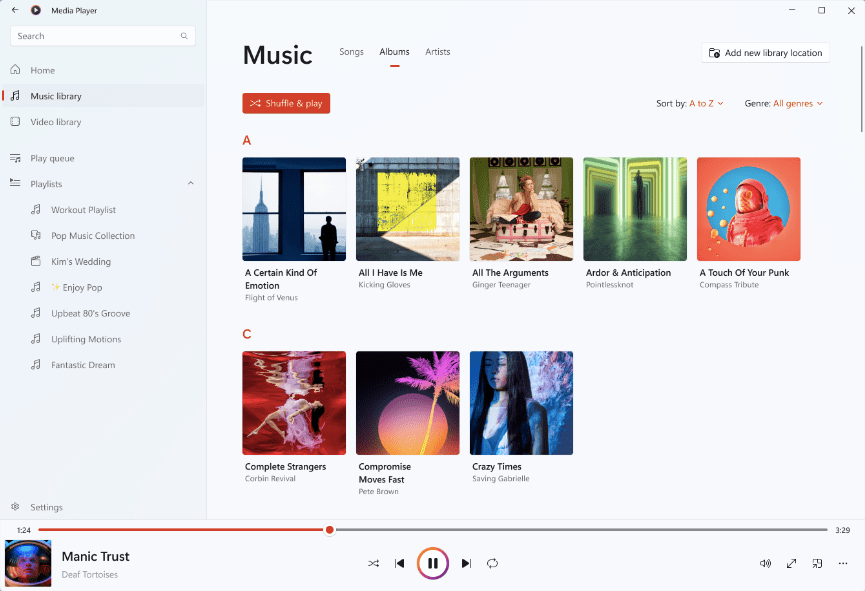The image displays a Windows device screen showing a media player application. On the left pane, the application header reads "Media Player." Below it is a white search bar labeled "Recent Search." The left sidebar contains several navigation options including Home, Music Library (which is currently highlighted), Video Library, Play Queue, and Playlist. Under the Playlist section, various playlists are listed: Workout Playlist, Pop Music Collection, Kim's Wedding, Enjoy Pop, Upbeat 80s Groove, Uplifting Motions, and Fantastic Dream.

The central section of the player displays content from the Music Library. It includes tabs for sorting music by Songs, Albums, and Artists. On the right side of this section, there is a button labeled "Add New Library Location." Below this, there is a prominent orange button that reads "Shuffle and Play." Next to this button, the music is sorted alphabetically from A to Z, and the genre filter is set to "All Genres."

Under the music sorted by the letter 'A,' the following tracks are listed:
- "A Certain Kind of Emotion" by Flight of Venus
- "All I Have Is Me" by Kicking Gloves
- "All the Arguments" by Ginger Teenager
- "Ado and Anticipation" by Pointless Nuts
- "A Touch of Your Punk" by Campus Tribute

Tracks under the letter 'C' include:
- "Complete Strangers" by Coping Revival
- "Compromise Move Fast" by Pete Brown
- "Crazy Time" by Saving Gabrielle

At the bottom of the playlist, "Manic Trust" by Deaf Tortoises is currently playing, and the player controls are visible. These include a play icon, shuffle icon, next and previous track icons, and a repeat icon. In the bottom right corner, there are additional controls for volume, maximizing the window, mini playback mode, and an options button.